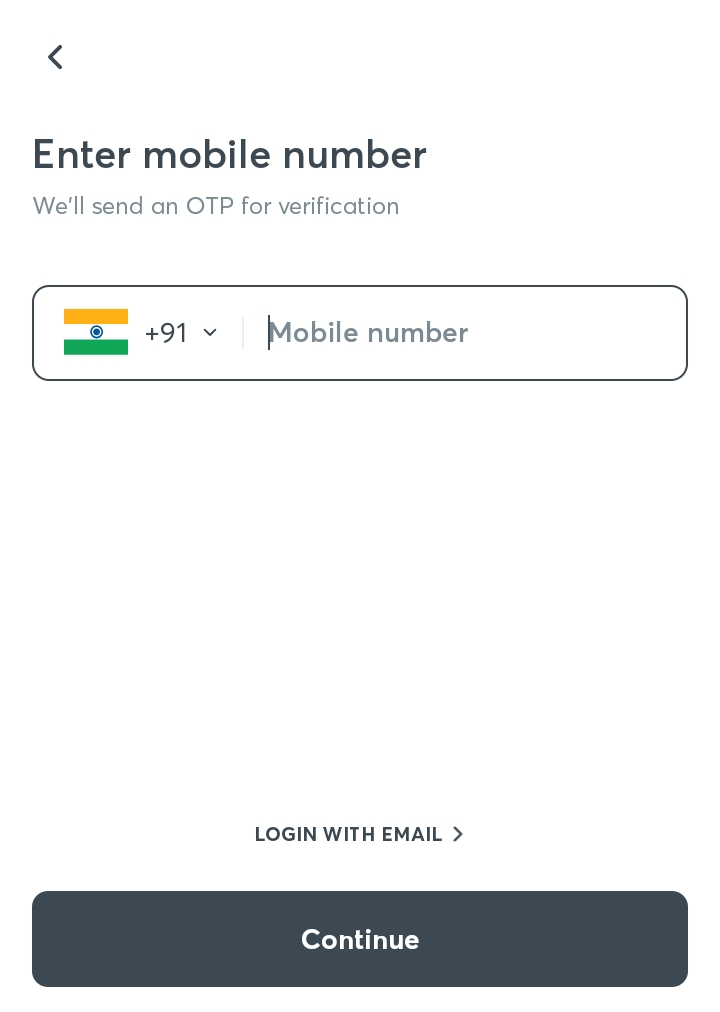This screenshot captures a mobile interface designed for user authentication through a mobile number. At the top, the interface prompts the user with the instruction "Enter mobile number" in black text, followed by a smaller note stating, "We'll send an OTP for verification." Positioned beneath this instruction is a rectangular input field. To the left of this field, there's an icon displaying the tricolor flag of India, which consists of horizontal bands of orange, white, and green, with a blue wheel featuring 24 spokes centered on the white band. Adjacent to the flag is the country code "+91," indicating that the user should input an Indian mobile number.

The main portion of the screen is predominantly blank, offering uncluttered white space that directs focus to the essential input sections. Towards the bottom-center of the screen, there is an option labeled "Log in with email." Just below this option, a gray button with the word "Continue" in white text appears, inviting the user to proceed with the verification process.

The overall design is minimal and user-friendly, ensuring clarity and ease of use by limiting the visible text and graphics to essential elements pertaining to the mobile number input and authentication process.